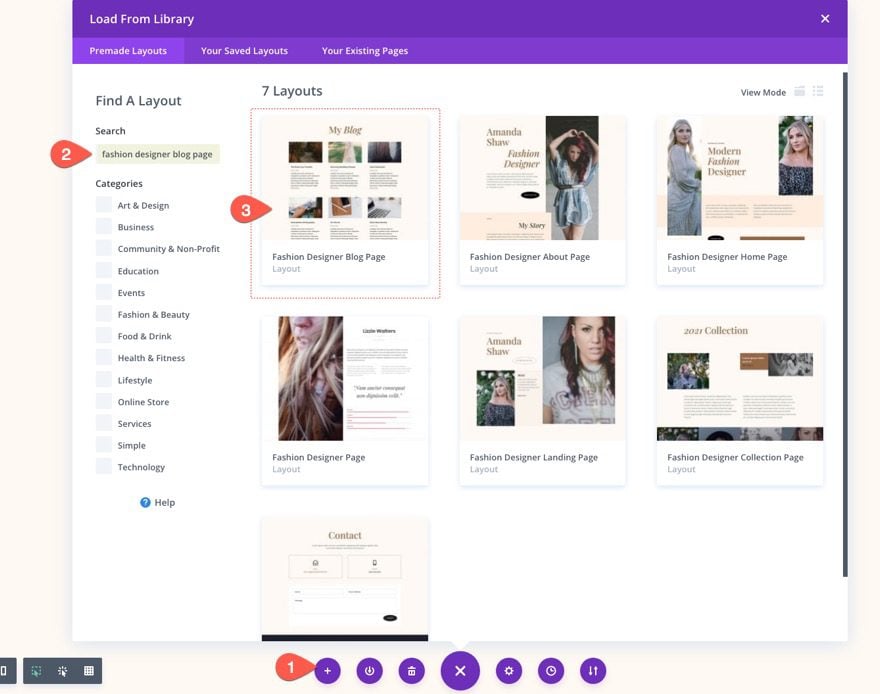The image features a dark purple header with the text "Load from Library." Below this header, there are tabs labeled "Pre-made Layouts," "Your Saved Layouts," and "Your Existing Pages." The left sidebar contains a search option labeled "Find a Layout" with a sample search query "fashion designer." Below the search bar, categories such as "Bling Page," "Block Page," and an indeterminate option "I Don't Know" are listed. A red arrow marked with the number "2" points at these categories. Underneath, there are further categories listed: "Art and Design," "Business," "Community and Non-Profit," "Education," "Fashion and Beauty," "Food and Drink," "Health and Fitness," "Lifestyle," "Online Store," "Services," and "Technology."

To the right, there is a box labeled "Seven Layouts" with a red arrow marked "3" pointing towards it. Additionally, at the bottom, a random purple circle with a "1" in the center is also indicated by another red arrow. This complex layout appears to guide the user through various sections and categories within a design or layout selection interface.